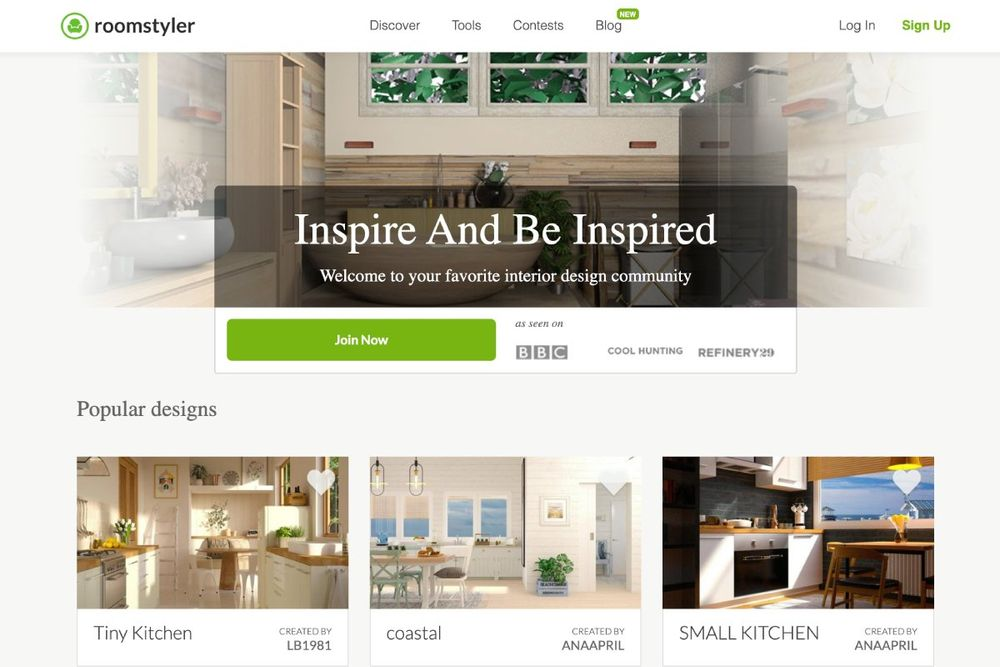In the upper left corner, there is a green-outlined circle with a green element inside it, labeled "Room Styler." Adjacent to it are menu options labeled "Discover," "Tools," "Contents," and "Blog," with the "Blog" label highlighted by a green rectangle that says "New." To the right, it has "Login" in standard text and "Sign Up" highlighted in green.

The main image displays a room with large windows at the back, overlaid with a semi-transparent black rectangle that reads "Inspire and Be Inspired. Welcome to Your Favorite Interior Design Community." Below this message is a white rectangle outlined in grey, containing a green button labeled "Join Now." Underneath, there is text stating "As Seen On," followed by grey squares with logos for "BBC," an indistinct second logo, and "Refinery 29."

Further down, the section titled "Popular Designs" showcases three pictures of kitchen designs. The first image is labeled "Tiny Kitchen," created by LB1981. The next image is titled "Coastal," created by ANAAPRIL. The final image is named "Small Kitchen," also created by ANAAPRIL.